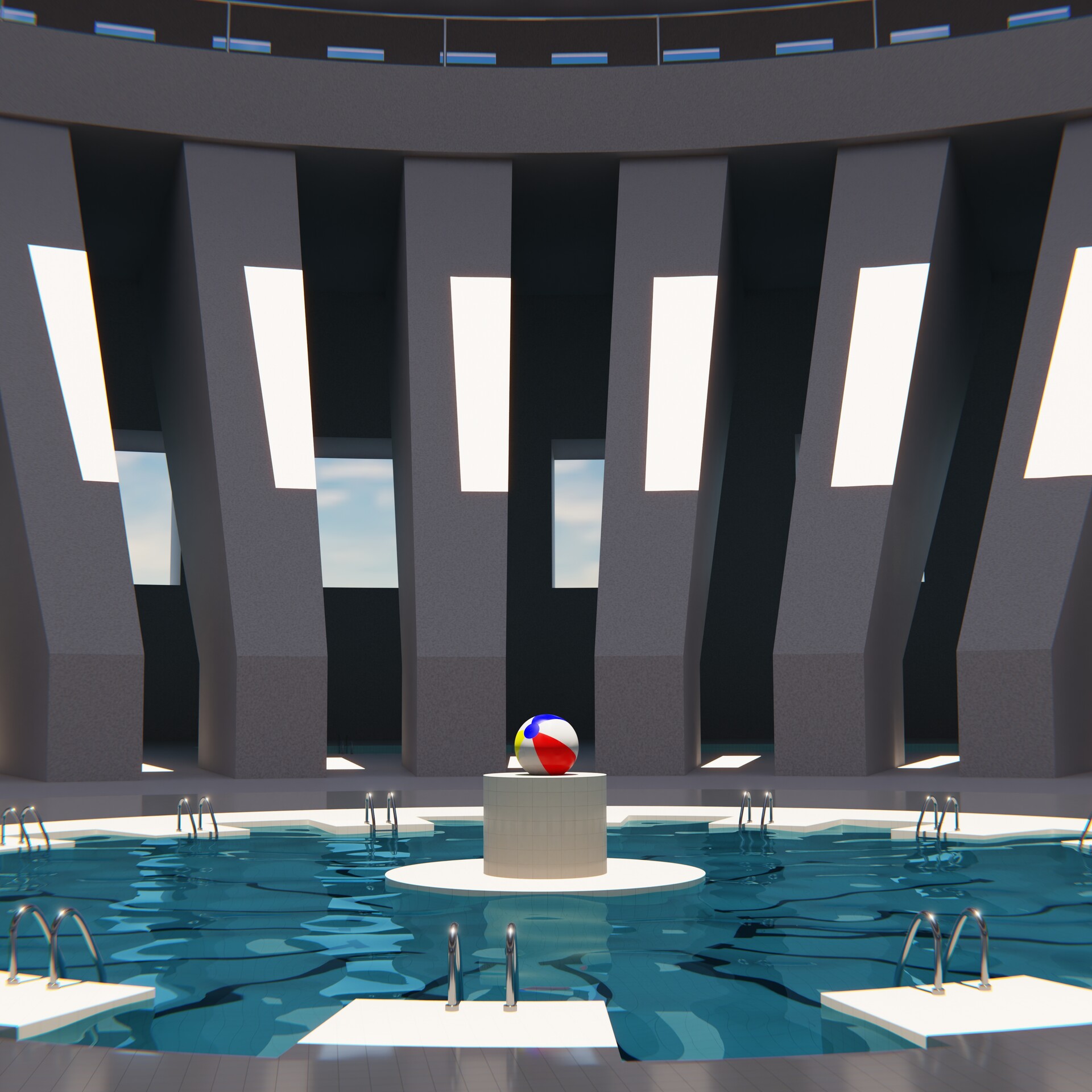This detailed computer-generated image depicts an indoor, circular swimming pool with a strikingly clean and well-lit environment. The pool features a central pedestal topped by a vibrantly colored beach ball, painted in alternating stripes of red, white, blue, white, yellow, and white. Surrounding the pool, white platforms are equipped with individual stainless steel ladders that provide access into the clear, blue water. Between these ladders are designated seating areas. Additionally, the pool contains lane markers that radiate from the perimeter toward the central pedestal, suggesting a structured design, possibly for a sport or game. The room itself is architecturally impressive, with tall, wide gray pillars that support a domed ceiling. Large windows between the pillars let in natural light and offer a view of the blue sky outside, while smaller dashed windows at the top add to the illumination. The overall scene combines functional elements with a visually appealing structure that emphasizes both elegance and utility.